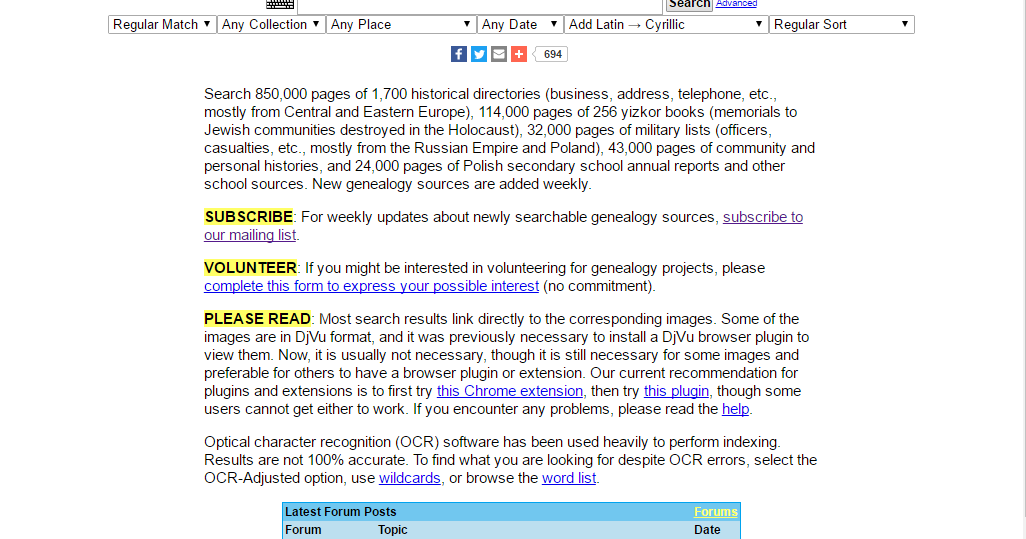This screenshot showcases a website with a clean, white background and black font. At the top of the page, there are several drop-down menus arranged from left to right. The menus are labeled as follows: "Regular Match," "Any Collection," "Any Place," "Any Date," "Add Latin," followed by an arrow which expands to show "Cyrillic," and "Regular Sort."

Beneath these menus are four small icons representing social media and sharing options. From left to right, these icons are for Facebook, Twitter, Email, and a plus sign. Emanating from the plus sign is a speech bubble containing the number "694".

Further down the page, a block of text in black font reads: "Search 8,500 pages of 1,700 historical directories, business address, telephone, etc., mostly from Central and Eastern Europe; 114,000 pages of 256 Yizkor books, memorials to Jewish communities destroyed in the Holocaust; 32,000 pages of military lists, officers, casualties, etc., mostly from the Russian Empire and Poland."